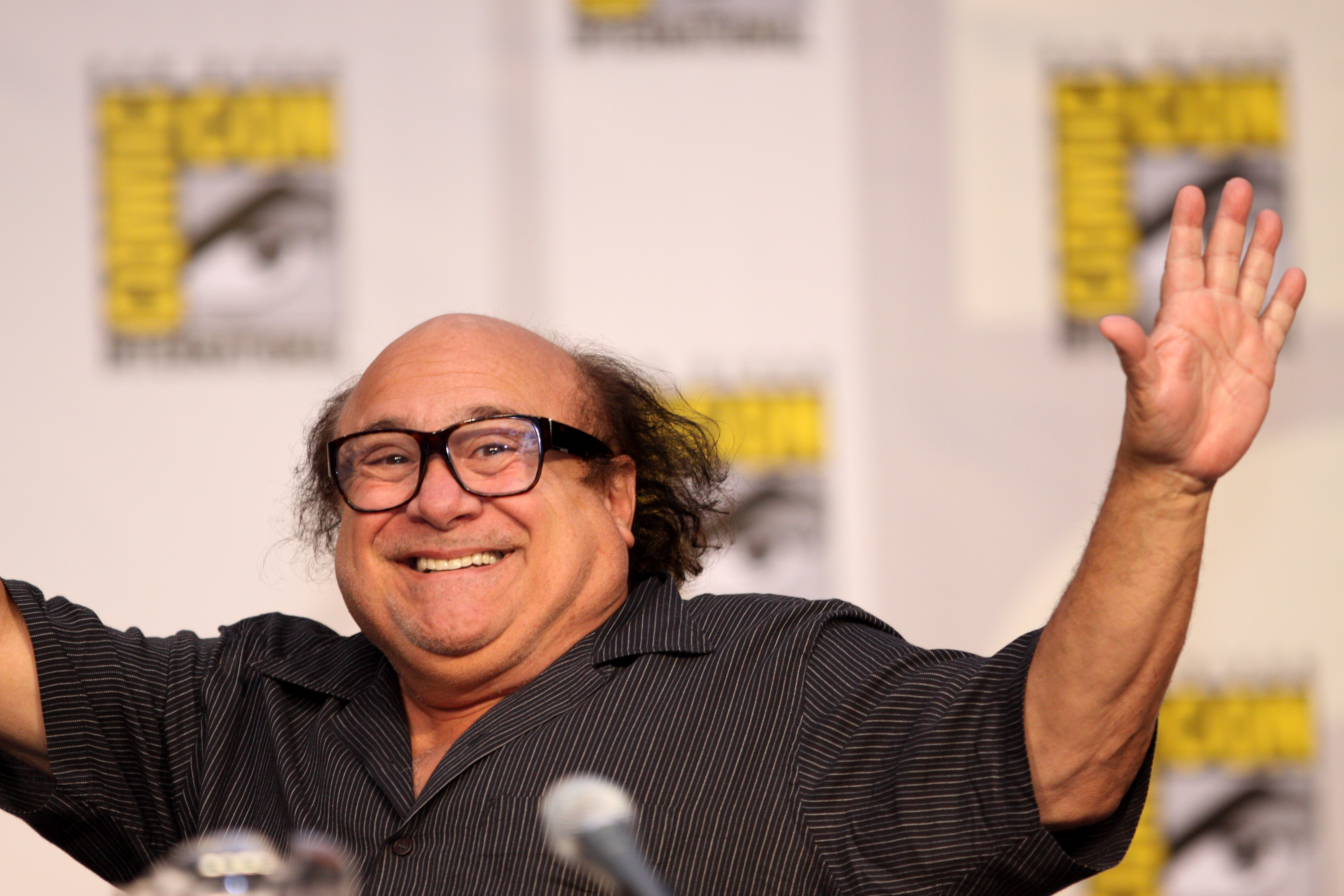In this horizontally oriented and somewhat blurry image, actor Danny DeVito stands in front of a microphone on a podium at Comic-Con. Behind him is a white wall adorned with square banners featuring the Comic-Con logo, which includes yellow lettering and an eye emblem. DeVito, recognizable by his bald head and longer brown hair at the back, is smiling broadly, showing his teeth. He wears black glasses with thick side rims and is dressed in a black striped short-sleeved button-down shirt. Both his hands are raised, as if he's waving, but due to the photo's framing, only his left arm is fully visible with his palm outstretched.